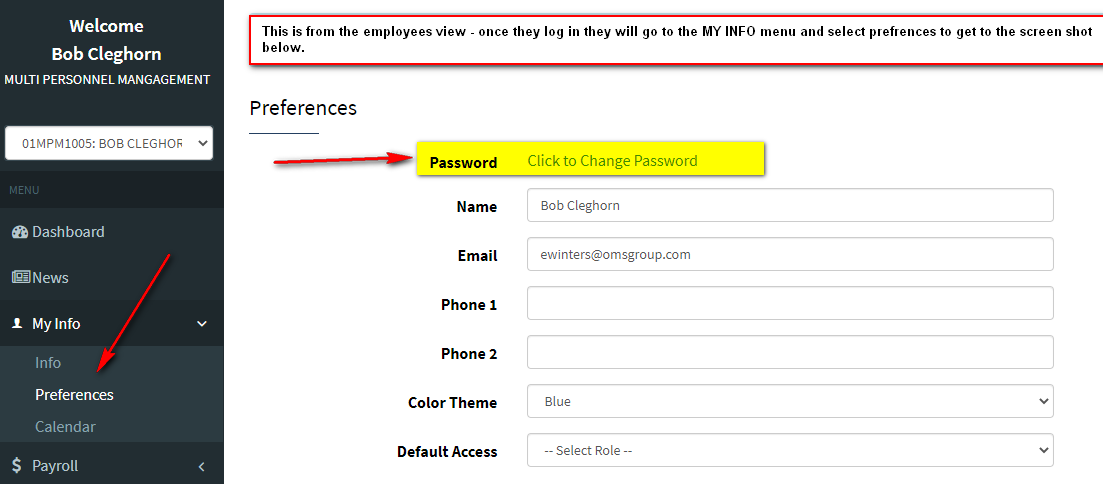Title: Detailed Employee Dashboard Interface for Learning Purposes

Caption: The image depicts a detailed view of an employee dashboard interface designed for learning purposes. A black vertical navigation bar on the left includes various menu items: Welcome, Bob; CLEG; HORN; and Multi-Personnel Management. Below, a drop-down menu labeled 'Bob' reveals Bob's ID (01MPM1005) and last name, both displayed against a white background. Other menu options listed are Menu, Dashboard, News, My Info, Info, Preferences, Calendar, and Payroll. A red arrow points specifically to 'Preferences,' indicating its importance. When 'Preferences' is selected, an arrow points to the 'Password' section, which is highlighted in yellow and advises to "Click to change password."

Above the main content, a red rectangle frames an instructional note: "This is from the employee's view. Once they log in, they will go to the My Info menu and select Preferences to get the screenshot below." The subsequent screenshot displays editable fields such as 'Name,' 'Email,' 'Phone One,' and 'Phone Two,' as well as drop-down menus for 'Color Theme' (set to blue) and 'Default Access' (for selecting roles). This detailed view ensures employees understand how to navigate and update their personal preferences efficiently.